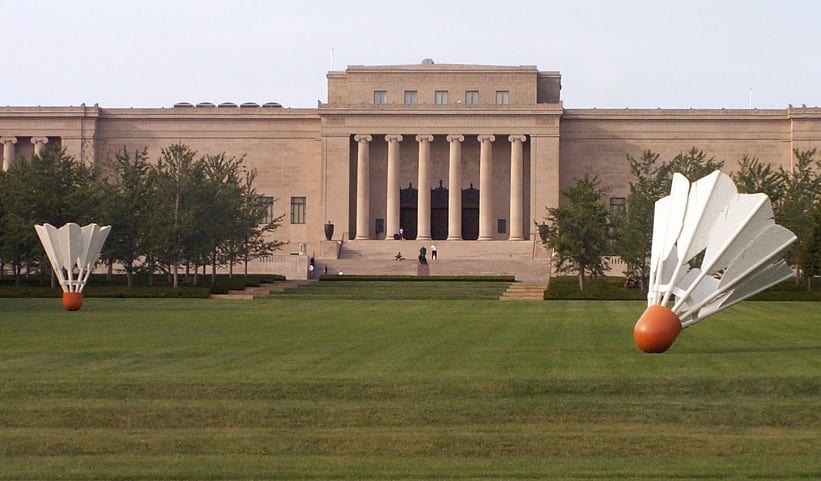In the image, there is a sprawling open field of freshly cut green grass occupying the bottom half, dotted with two massive sculptures shaped like badminton shuttlecocks. One shuttlecock, positioned on the far right, is embedded in the ground at a 45-degree angle with its white feathers and orange tip prominently displayed. The second shuttlecock stands upright in the middle left of the image. Both sculptures are set against a backdrop of leafy trees on either side of the field.

Dominating the center is a grand building featuring tall pillars, numerous steps, and dark windows at the top. The building has a tan or brownish exterior, evoking a sense of historical or significant architectural importance. The structure is framed by additional trees on both sides, reinforcing the outdoor setting. The upper section of the image reveals a clear blue sky, which enhances the vivid colors of the scene: the green of the grass, the white and orange of the shuttlecocks, and the tan of the building. The unconventional placement of the shuttlecock sculptures in such a formal setting adds an intriguing, almost surreal element to the photograph.